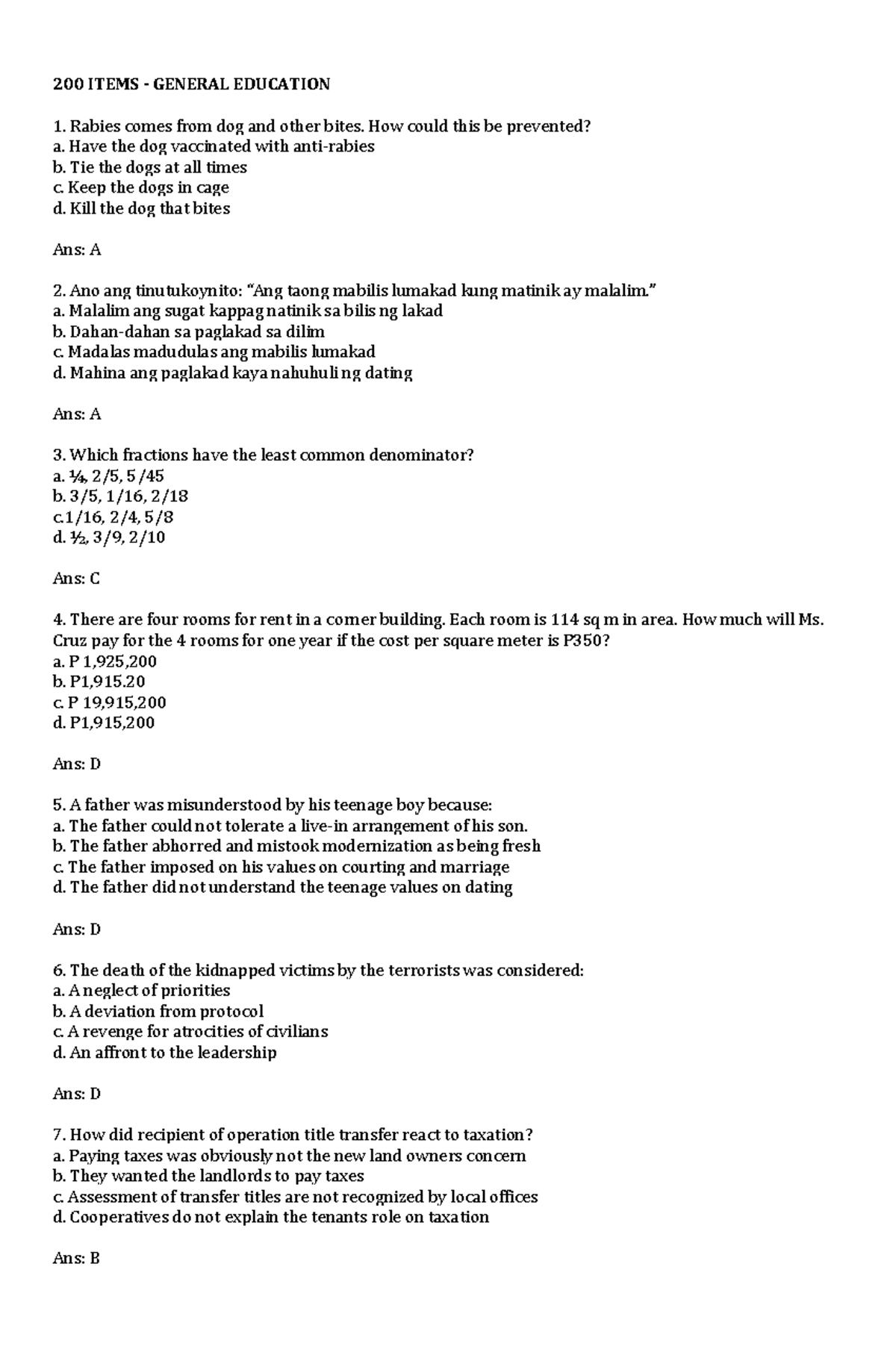This screenshot captures a detailed answer key for a general education test featuring 200 items. The text is presented in a list format, displaying each question alongside multiple-choice answers and indicating the correct one for each query.

At the top of the screenshot, the document title specifies "200 items, General Education." The first question reads, "Rabies come from dog and other bites. How can this be prevented?" and offers four possible options: A) Have the dog vaccinated with anti-rabies, B) Tie the dog at all times, C) Keep the dogs in cage, and D) Kill the dog that bites. The correct answer provided is A.

Interestingly, the second question diverges from the pattern, being written in a different language: "Ano, ang, tin, tuku, yanito, angtao, mabulis, lumakad, kung, matinik, ay, malalim." The options are similarly foreign, and the correct answer here is A.

The caption also notes that the rest of the questions revert back to English. For instance, the third question is, "Which fractions have the least common denominator?" with the correct answer listed as C.

The last notable question highlighted is number seven, asking, "How did the recipient of operation title transfer react to taxation?" The screenshot suggests that this document continues with a variety of questions, all provided with the correct answers, making it a comprehensive answer key for a general education test.